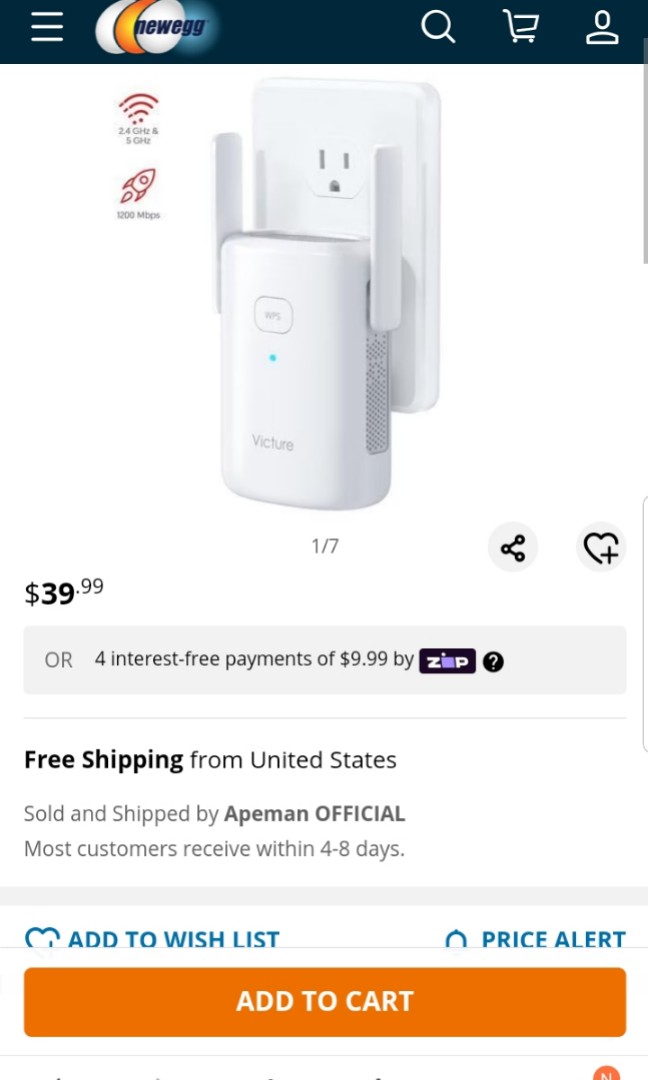This image is a screenshot of a Newegg webpage viewed on a tablet, showcasing a Wi-Fi range extender. The dark bluish-black menu bar at the top features icons in white: a hamburger menu on the left, a magnifying glass for search, a shopping cart, and a user profile icon.

Central to the screenshot is the product image of the Wi-Fi range extender, identified as the VICTURE model. The device is a compact, white plug-in unit equipped with two Wi-Fi antennas and a green indicator light marked "WPS." It supports both 2.4 GHz and 5 GHz frequencies and boasts speeds up to 1200 Mbps, evidenced by a small icon of a rocket and Wi-Fi symbols.

The product is highlighted as available for $39.99, with an alternative option of four interest-free payments of $9.99 through ZEP. Free shipping is provided from the United States, with delivery typically occurring within four to eight days. The product is sold and shipped by Ape Man Official.

Additional details on the page include options to share or mark the item as a favorite, view seven different images of the product, and add it to a wish list or price alert. The page clearly indicates that it is geared towards users considering the purchase of a Wi-Fi range extender.